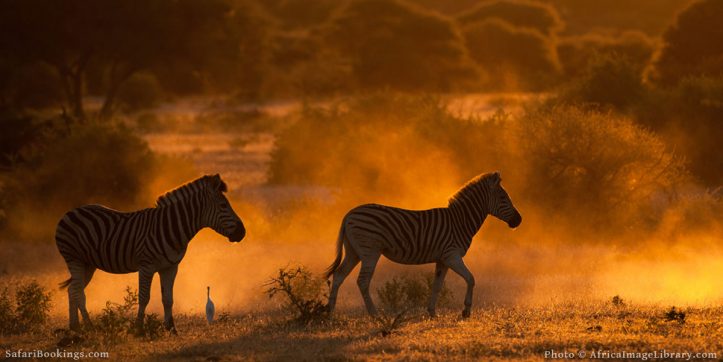This is a detailed, color photograph capturing two zebras standing in profile, facing right in the Serengeti, Africa. The scene is bathed in the golden-orange hues of a setting sun, casting a warm glow over everything. The ground beneath the zebras is grassy, while the background features red dust clouds, tall trees, and various bushes, suggesting a recent disturbance, possibly from a passing vehicle off-frame. A small white bird stands between the two zebras, adding to the sense of life and movement. The sky shows dark clouds, enhancing the dramatic lighting. Visible at the bottom of the image are two translucent white watermarks: "photo copyright AfricanImagesLibrary.com" and "safaribookings.com," marking the photograph's origin and usage.